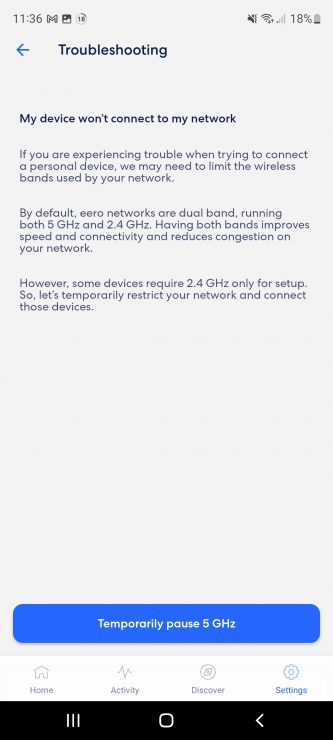Here is the revised and detailed caption for the image:

---

The image is a mobile device screenshot displaying various icons on the status bar at the top. The time is shown as 11:36, accompanied by a mail icon, a Google Photos icon, and a calendar icon. On the right side of the same row, there is a vibrate icon, a strong Wi-Fi signal indicator, a full cellular signal icon, and an 18% battery level icon.

The main section of the screen features a page titled "Troubleshooting" in large text. Beneath the title, a horizontal line separates it from the content below. The first line of the content is in bold font, reading "My device won't connect to my network."

Following this, there are three unbolded paragraphs that provide troubleshooting steps. The text reads:

"If you are experiencing trouble when trying to connect your personal device, you may need to limit the wireless bands used by your network. By default, Eero networks are dual-band, running both 5GHz and 2.4GHz. Having both bands improves speed and connectivity, and reduces congestion on your network. However, some devices require 2.4GHz only for setup. So, let's temporarily restrict your network to connect those devices."

At the bottom of the page, there is a prominent blue button with white text that says "Temporarily pause 5GHz." Below this button, there is a navigation bar with icons for Home, Activity, Discover, and Settings.

---